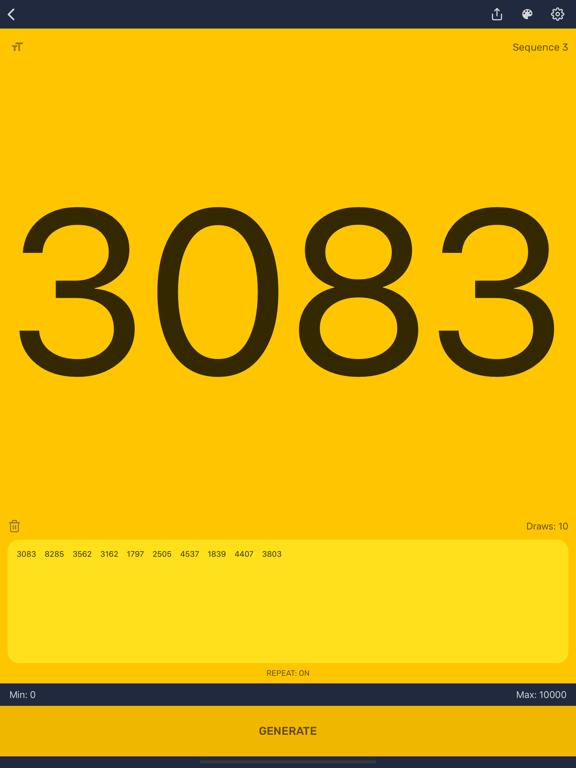The screenshot depicts a computer interface featuring a distinct dark yellow background with the prominent number "3083" in the center. At the top of the interface is a black bar containing a backward arrow on the left and icons for download, a camera, and settings on the right. Below the black bar is an area labeled "sequence 3" in smaller text. Beneath the large number "3083", there is a column of smaller numbers on a light yellow background, including 3083, 8285, 3562, 3162, 1797, 2505, 4537, 1839, 4407, and 3803. Below this column is another section labeled "repeat: on." Further down, a blue bar stretches across the interface with "minimum: 0" on the left and "max: 10,000" on the right. Below this, there is a dark yellow strip with the word "generate" in the center. At the bottom of the image, there is an additional, thinner blue bar.